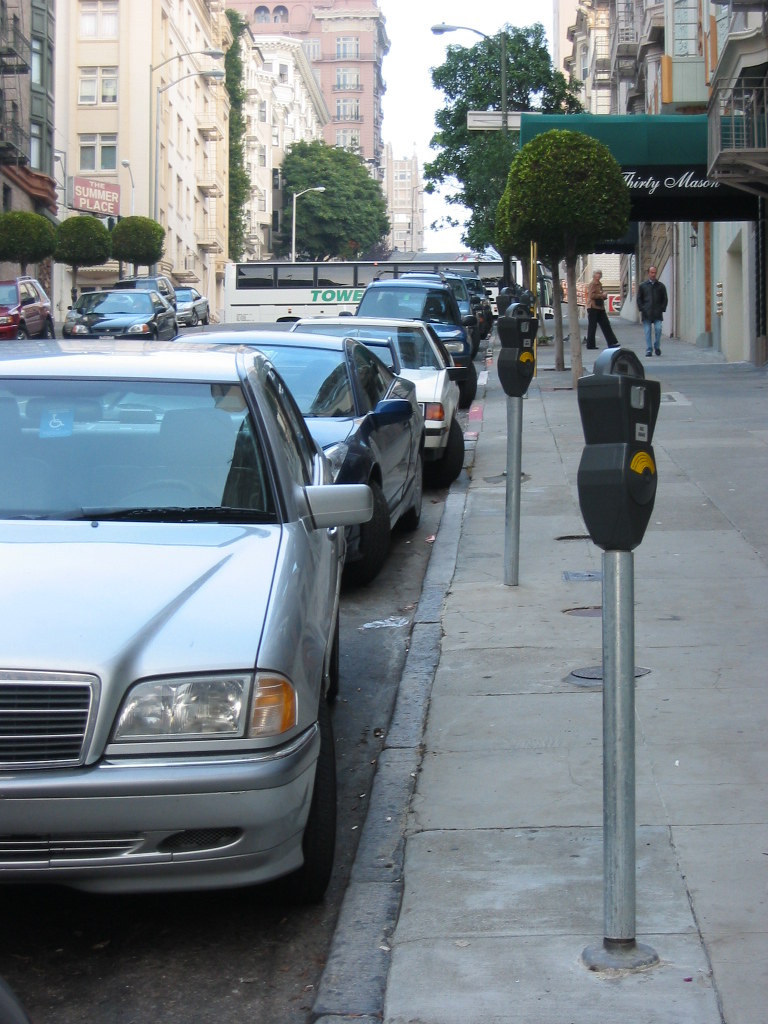This vibrant color photograph captures a bustling city street scene, possibly set in San Francisco, characterized by its hilly terrain. The composition is parallel to the street, showcasing several five to seven-story residential-looking buildings lining both sides. Prominent in the image is a wide concrete sidewalk with green awnings jutting out from the establishments; one such awning, labeled "30 Mason," suggests the presence of a business, perhaps a hotel or an apartment building entrance.

The street is populated with numerous slightly dated cars, likely from the late 1990s or early 2000s, parked alongside parking meters that dot the sidewalk. The presence of green trees in potted areas adds a touch of nature to the urban setting. Up the hill, the street scene continues with visible intersections, including a shop at the corner adorned with a red sign reading "The Summer Place." A bus bearing partial letters "T-O-W-E," presumably heading towards a tower, traverses the intersection. The tallest building visible up the hill is pink, further adding to the city's eclectic architectural mix. The overall scene captures the dynamic essence of a vibrant, urban neighborhood.